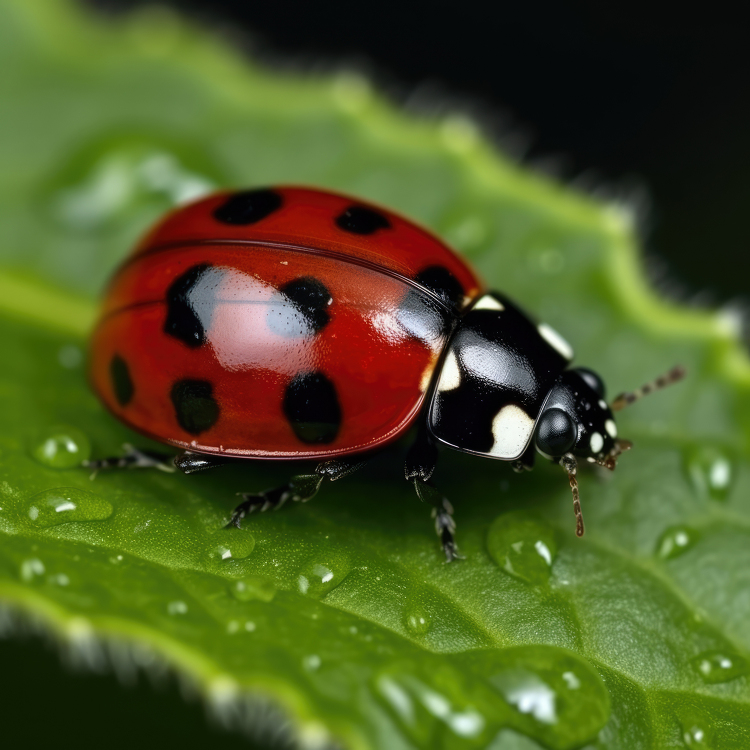This striking image showcases an extreme close-up of a ladybug perched on what appears to be a holly leaf. The ladybug, occupying the center of the frame, displays its deep red wings adorned with shiny black spots. Its glossy neck is mostly black with small white dots, leading up to its head, which features large black eyes, black dots near the nose, and small antennae. The ladybug's black legs, detailed with small spines, contribute to its crawly appearance. The texture of the leaf, hinted by the pointed edges and tiny hair-like structures, is accentuated by numerous droplets of water. The background is almost entirely black, making the vivid colors of the ladybug and the leaf stand out prominently, creating an almost surreal visual effect. The sharp focus on the ladybug, coupled with the slight blur of the leaf, adds depth to this mesmerizing image.